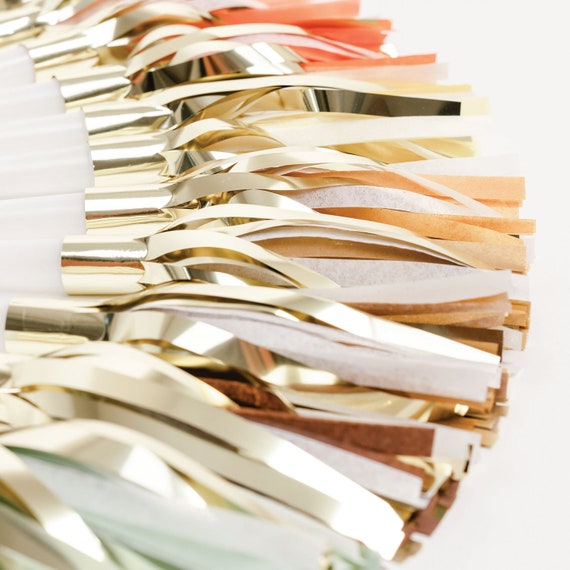The image features a collection of objects resembling cheerleader pom-poms, neatly arranged in a semi-circle from the bottom left to the top left against a white background, possibly a table. Each pom-pom has a white handle adorned with metallic gold wrapping at the top. From the handles, vibrant ribbons burst out, with hues of red, gold, white, pale orange, apricot, and brown, creating a lively and colorful display. Notably, all the handles appear identical, except for one situated in the middle left, which seems to have a black mark on it, perhaps due to lighting. The overall effect is that of festive, eye-catching decorations ready to be shaken to add visual excitement, much like traditional cheerleader pom-poms.